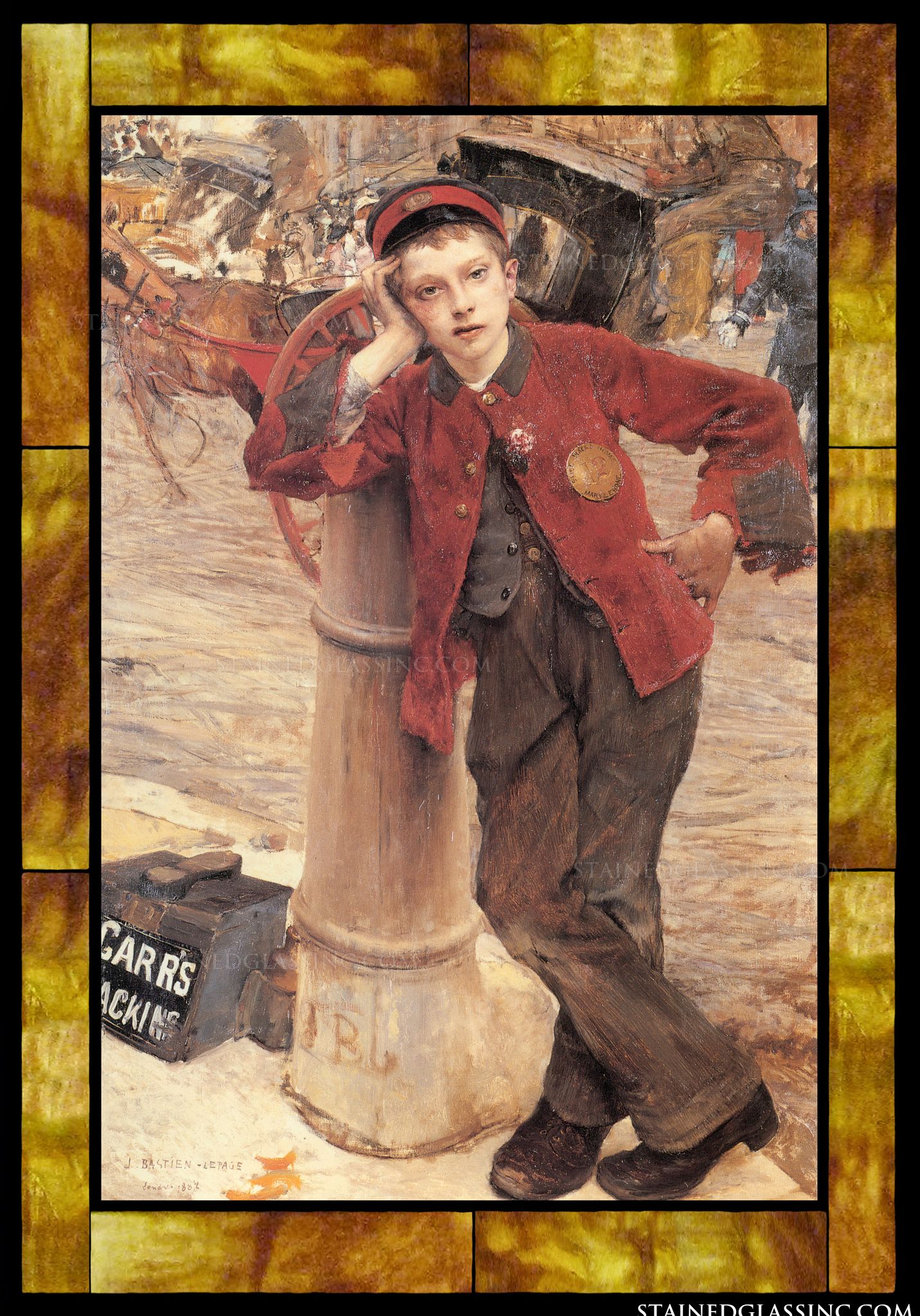An evocative, old-fashioned photograph likely dating back to the 1800s features a young boy in period attire. The image is bordered by a golden-brown, swirling frame, intermittently divided by slim black lines which give it an antique elegance. Nested within this frame is a second picture, outlined by a thin black line, creating an effect reminiscent of a picture-in-picture frame.

The boy leans against what appears to be a large wheel with a thick stump or pole beside him, adding a rustic charm to the scene. He is dressed in a striking red jacket, accented with a brown collar and brown details at the sleeves. The jacket is buttoned at the top, revealing a brown or gray vest beneath. The boy wears long, brown pants, with his legs crossed and one foot bent outward. His shoes are a matching shade of brown.

He gazes directly at the camera, wearing a black cap with a red band and a round metal embellishment on the front of his jacket, possibly flowers near the button. The ground beneath him is brown, and an old-style item, potentially a shoeshine stand, is partly visible.

The background is filled with a scene of apparent clutter, creating a sense of disorder; various items are piled up, contributing to the chaotic backdrop. To the far right, a figure that resembles a police officer dressed in gray is partially visible, his face and right side obscured.

At the very bottom of the photograph, partially cut off, is the text "stainedglass.com" in white atop a black trim, lending an additional layer of mystery to this historical snapshot.